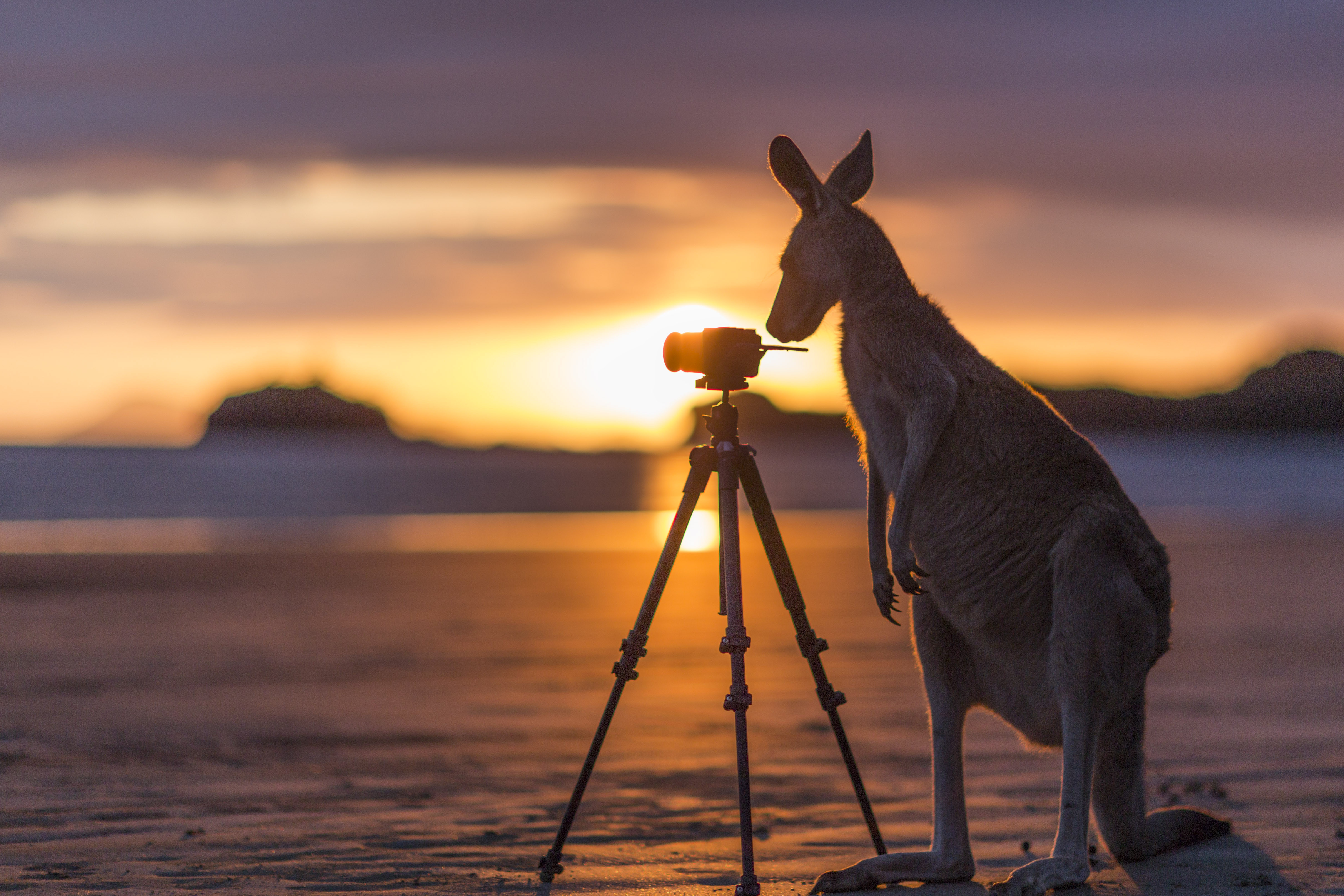This humorous outdoor photograph captures a whimsical scene at sunset. In the sandy setting with no vegetation, a kangaroo stands silhouetted against the glow of the sun. Positioned towards the right, the kangaroo, with its large ears, big legs, and slender front limbs, leans in curiously towards a camera mounted on a black tripod. Its nose almost touches the camera, suggesting a comedic moment as if it's preparing to snap a picture. The background features a vivid gradient sky, transitioning from purples at the top to vibrant oranges and yellows near the setting sun, which sits directly behind the camera, casting a strong silhouette. To the left, a dark mass resembling a mountain is visible, while to the right, there are outlines of smaller hills. The horizon line conveys a faint impression of water or a stream, adding to the depth and visual interest of the composition. The entire scene is bathed in the warm, glowing hues of twilight, enhancing the enchanting and playful nature of the image.